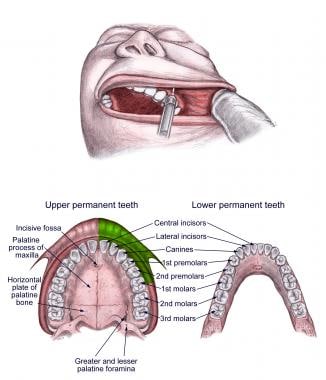The illustration appears to be from a dental textbook or instructional guide, featuring detailed images and labeling. The top portion of the illustration depicts a cartoon-style drawing of a man's face viewed from below, showing his mouth being held open by gloved fingers while a needle, likely administering Novocaine, is injected into his upper gums. This part of the image highlights a typical dental procedure. Below this, the image transitions into a detailed diagram of the teeth. The lower portion consists of two labeled diagrams: one for "upper permanent teeth," which has a green-shaded section, and another for "lower permanent teeth." Both diagrams use a palette of black, red, pink, and green, with each tooth distinctly labeled as incisor, canine, premolar, first, second, and third molar. The illustrations are comprehensive, with an emphasis on both the upper and lower jaw, providing a clear, educational view of the dental anatomy.